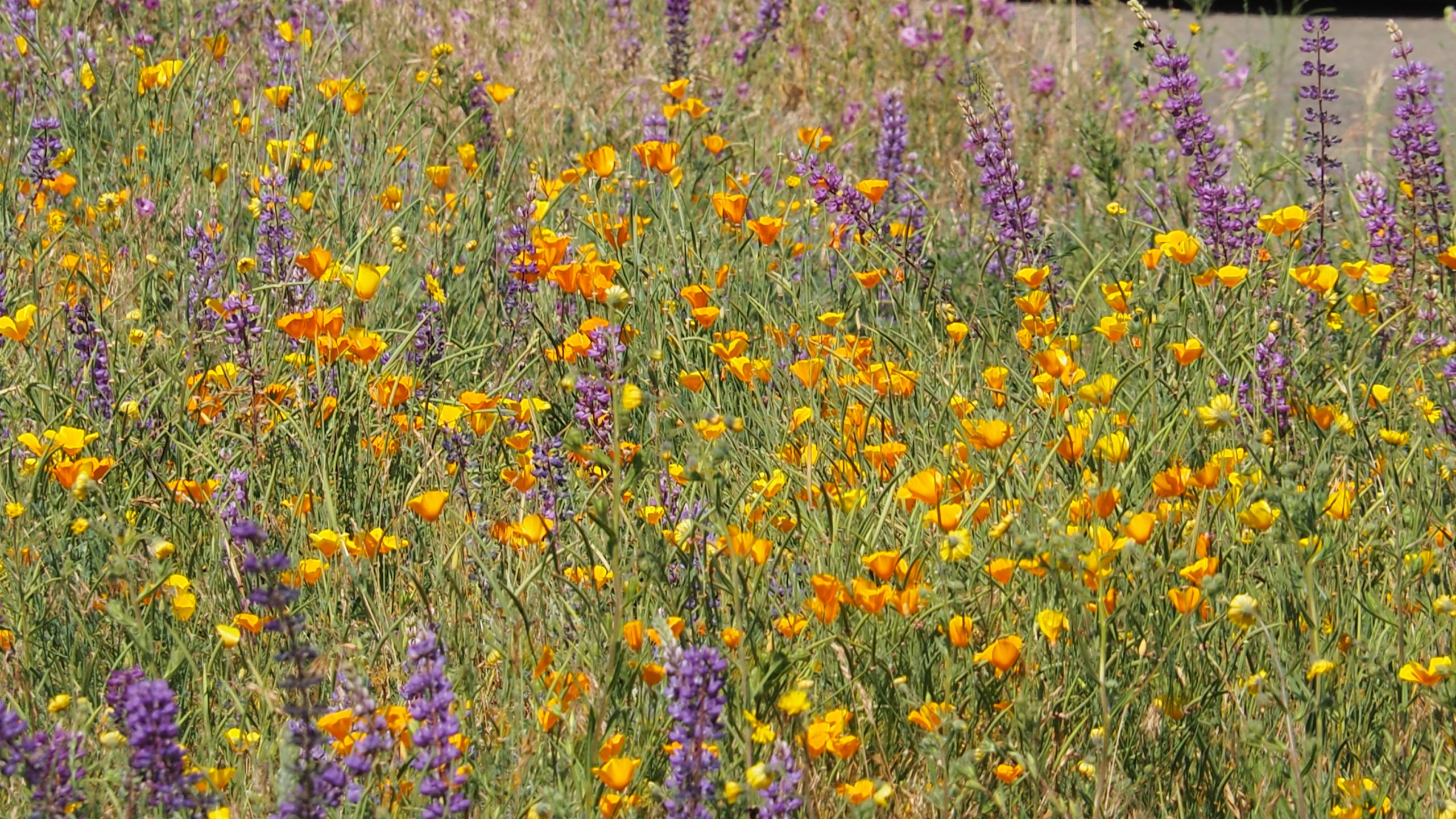This photorealistic image features a vibrant field brimming with wildflowers under bright daylight. The scene is jam-packed with a plethora of flowers, prominently showcasing small orange-yellow blooms and taller, lavender-like purple flowers. These purple flowers, potentially a variety known as stachia, stand out with blooms branching from each side of a central stem. The flowers are interspersed across the entire field, creating a striking mosaic of colors. Intermixed with the blooms is an abundance of tall, lush green grass, which fills the spaces between the flowers, adding to the dense and lively atmosphere. The horizon is only visible at the top right-hand corner, emphasizing the sheer expanse of this wild and colorful prairie landscape. No trees, animals, or people are present, making the flowers and grasses the sole focus of this vividly detailed natural scene.